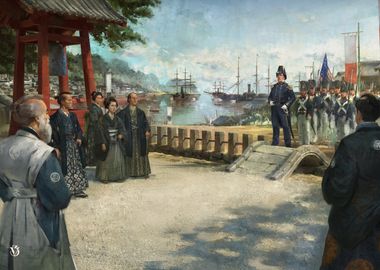The painting depicts a historical encounter on a coastal setting, possibly evoking themes of colonization or war. On the left side, there is a group of seven people, likely of East Asian origin, based on their traditional attire, which includes kimonos and samurai-like outfits. This group stands in front of a distinctly Japanese structure, with a reddish top, adding to the cultural context of the scene. The ground they stand on is beige, suggesting a courtyard or sandy landmass.

To the right, closer to the viewer, stands another individual dressed similarly in traditional attire, isolated from the main group. A small stone or wooden bridge, subtle in detail, connects these two sections of the painting.

In the background, a contingent of what appear to be American soldiers, identifiable by their blue jackets, white crisscrossing belts, and yellow trousers, is disembarking from several ships onto the shore. One soldier prominently carries the American flag, adding a sense of historical specificity. Leading this group is a commander dressed in a dark blue uniform, suggesting his leadership role.

The sky is painted a serene blue, with soft lines contributing to the realistic yet gentle aesthetic of the image. Behind the soldiers, a mix of vegetation and buildings provides further depth and context, completing the scene of cultural convergence and tension.